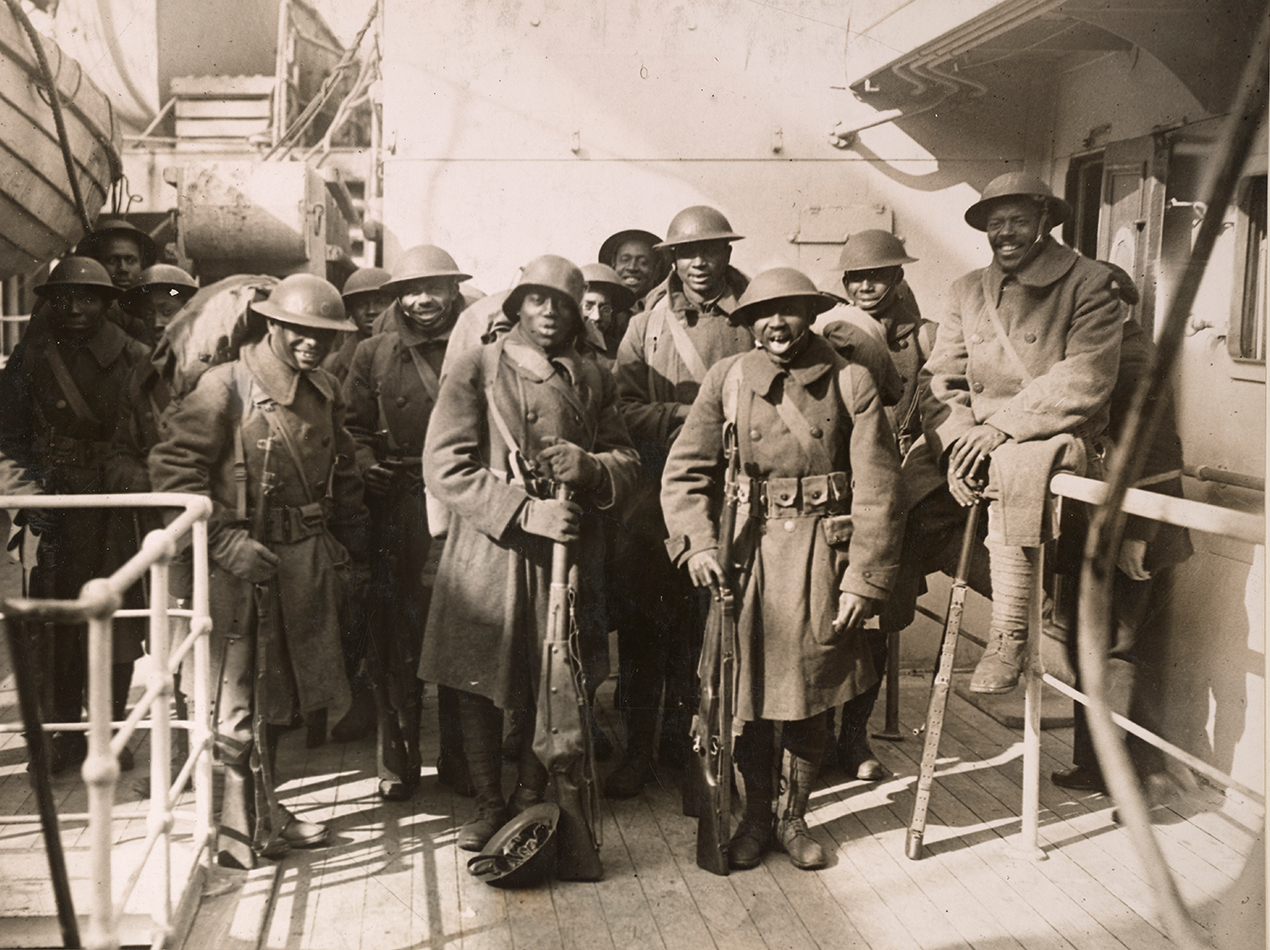This black and white photograph, tinged with sepia, showcases a group of 14 to 15 African-American soldiers from what appears to be the World War I era, standing on a wooden ship dock. The men are dressed in knee-length woolen peacoats, complete with munitions belts that have multiple pockets and compartments for carrying equipment. They are adorned with dome-shaped steel helmets and black boots, and their uniforms feature shoulder straps with bags. Most of the soldiers are standing, holding long rifles made of wood and steel. The front row of men grips their rifles by the barrel, with the butts resting on the ground, while one soldier, distinguished by his seated position on a railing, is part of the composition. A white fence-like rail and a metal-paneled wall form the backdrop for this poised and disciplined troop. The intricate details of their attire and the serene, yet authoritative stance of the men capture a moment of historical significance.